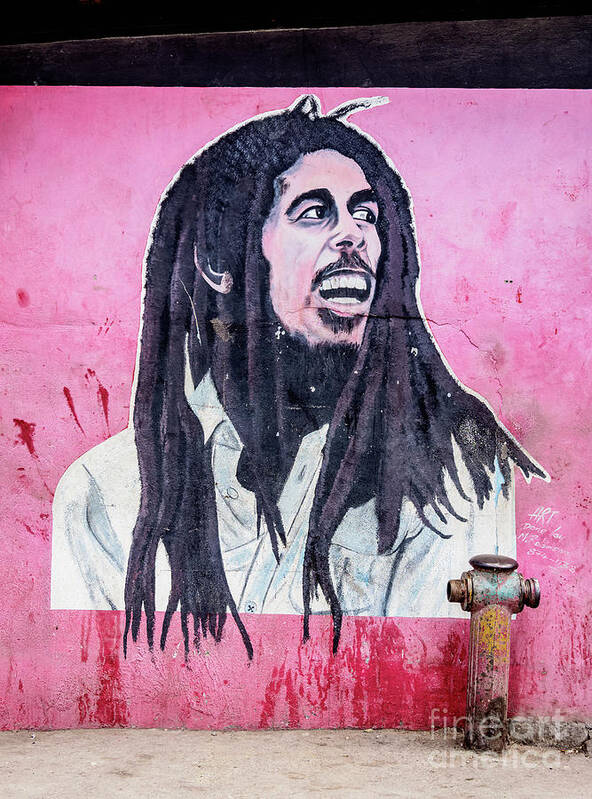The image features a vibrant mural painted on the side of a building, unmistakably credited to Fine Art America as indicated by a watermark in the bottom right corner. The mural predominantly portrays a man who bears a striking resemblance to Bob Marley, characterized by his long dreadlocked hair, dark eyebrows, beard, goatee, and mustache. He is attired in a white shirt, with his gaze directed towards the upper right side of the image. The mural artistically uses a pink background adorned with red splatters, creating a striking contrast. The figure in the mural is outlined in white, enhancing the focus on his expressive face, which reveals his open mouth showcasing very white teeth.

Notable elements within the mural include a metal object resembling either a hydrant or an old device, positioned near the man's left arm and seemingly splattered with paint. The ground in front of the mural is bare dirt. Adding an extra layer of depth, the artwork is signed by the artist with the initials "HRT," though further details written beneath the initials remain unreadable. The mural's placement on the building's exterior, adjacent to a visible sidewalk, firmly situates it within an urban landscape, making the painting not just an isolated piece but part of the living city environment.